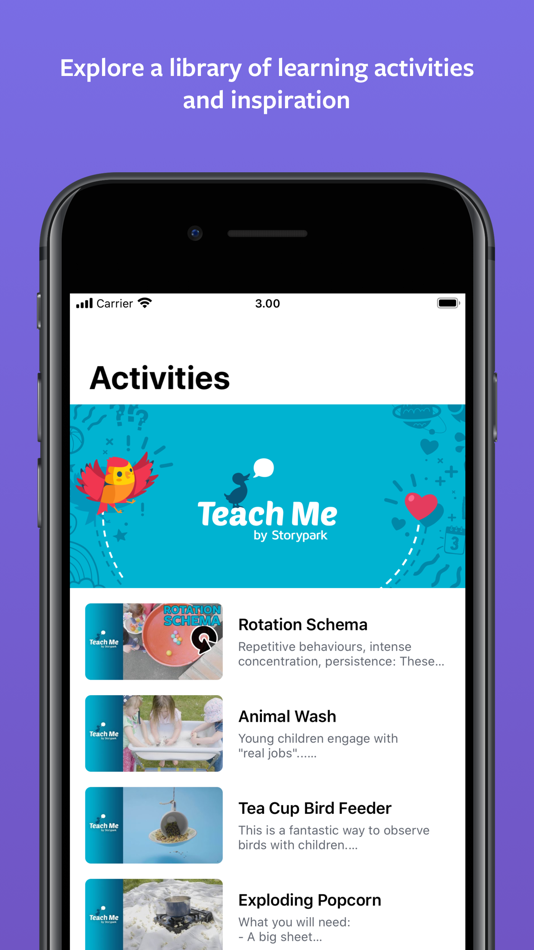A vertical rectangular box features a periwinkle blue background. At the very top, a caption in white letters reads, "Explore a library of learning activities and inspiration." Below this text sits an image of a black cell phone with a white ribbon across the top, inscribed with the word "Activities" in black. 

The phone's screen showcases a sample option from the library: a vibrant depiction on a light blue background. The illustration includes a colorful bird in shades of orange, red, and yellow, flying with its wings spread, accompanied by various playful symbols like a red heart, a yellow sun, a question mark, an exclamation point, a star, additional hearts, and a planet. At the center, white text proclaims, "Teach Me by StoryPark."

Below this central image, additional activity options are listed. The first option, "Rotation Schema," is in black text with a description in gray: "Repetitive behaviors, intense concentration, persistence." Next, "Animal Wash" in black text is described in gray as, "Young children engage with real jobs." Following this, "Teacup Bird Feeder" explains in gray, "This is a fantastic way to observe birds with children." Lastly, the activity "Exploding Popcorn" is listed in black text. Each of these options is accompanied by a brief blurb and a small image to their left, providing visual and textual details that would appeal to children.